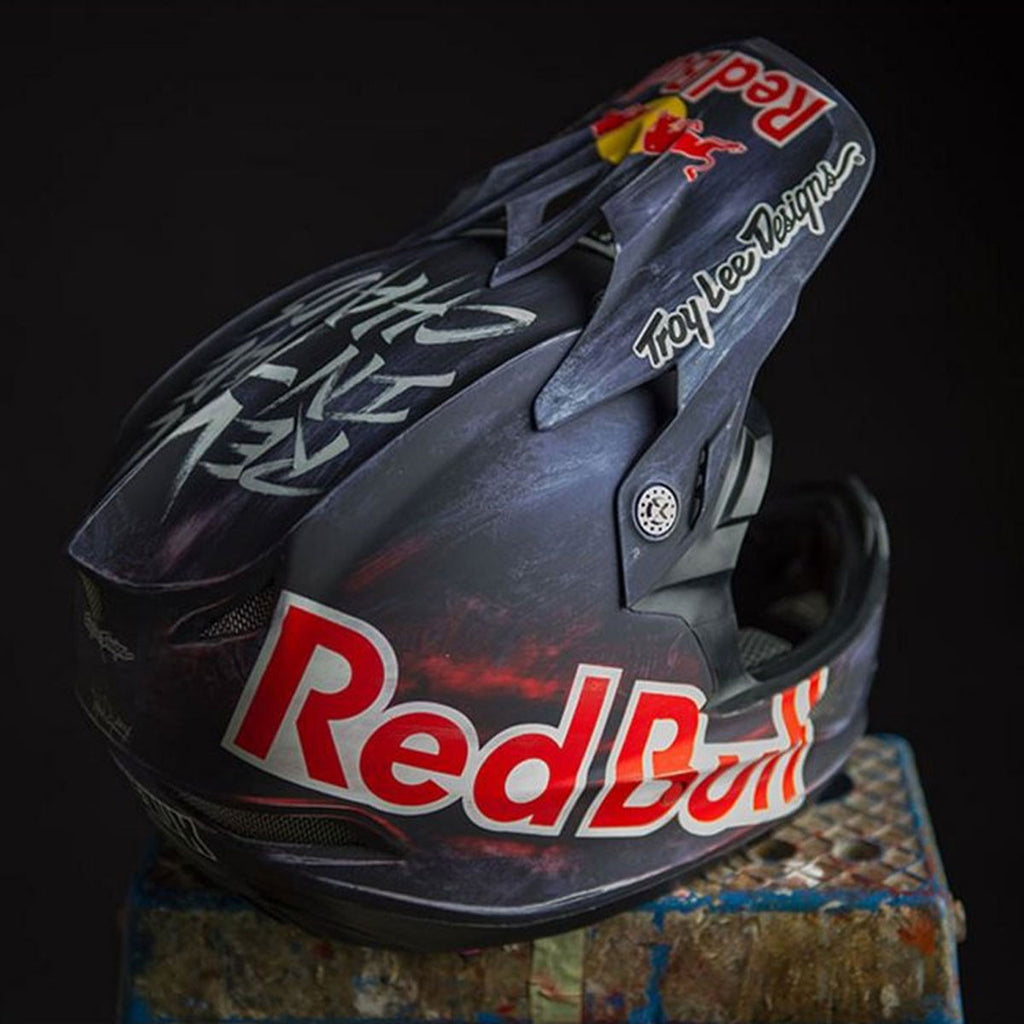This image features a worn, dirt bike-style motorcycle helmet predominantly in dark gray, accented with red splotches, sitting slightly tilted on the grooved surface of a vintage, golden-colored metal chest with intentional, stylistic holes. The helmet prominently displays the Red Bull logo in large red and white letters on both the visor, which is lifted, and the side. The visor itself features the iconic Red Bull graphic of two bulls charging with a white circle in between. On the right side of the helmet, "Troy Lee Designs" is written in cursive. Additionally, there is white text on the top of the helmet that reads "Revel in the Chaos," though it appears upside down. The chest, with its aged and painted look, adds a unique backdrop to the helmet, enhancing the image’s overall character and style.